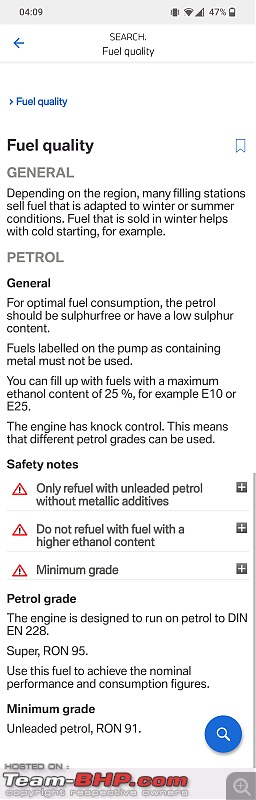This is a detailed screenshot from a smartphone displaying a search result within an app, possibly hosted by team.bhp.com, as indicated by a banner at the bottom of the page. The interface showcases a white background with black text, providing information under the main category "Fuel Quality," highlighted in blue at the top. The content includes a prominent header, "Fuel Quality," and a subheader labeled "General." The text elaborates on the various types of fuel available seasonally and specifies the appropriate fuel types for a particular engine. Additionally, the page contains important safety notes and detailed descriptions of petrol grades, guiding the user on the optimal fuel choices for their engine.